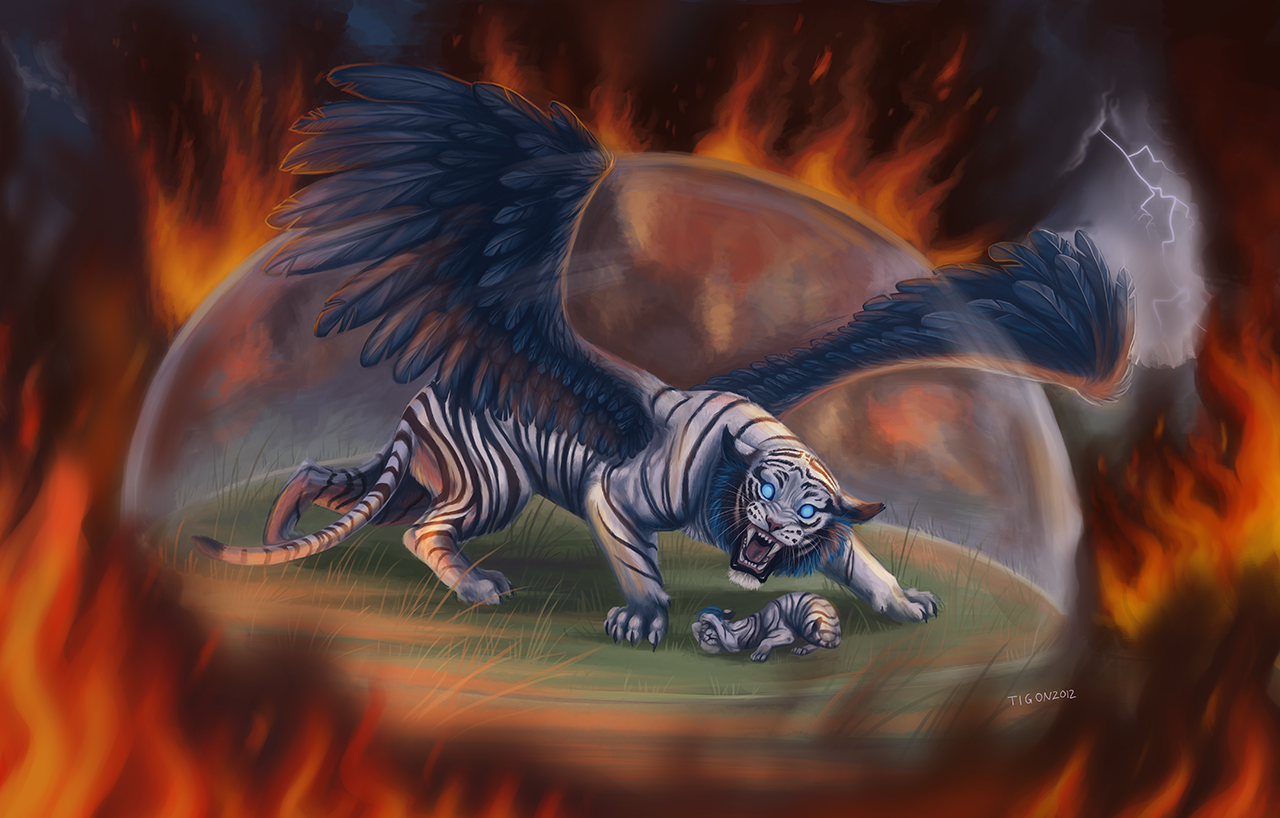The image is an intricate digital artwork resembling a poster, dominated by vivid, swirling flames in shades of orange, darker orange, and black. The flames encircle the central focus of the image, where a hybrid creature stands prominently. This creature has the body and bold stripes of a tiger, but with the distinctive black and white pattern of a zebra. Its intense blue eyes glow with a striking, arresting quality. The animal also possesses large, dark gray wings extending from its back, giving it a commanding and fierce appearance. The creature's mouth is open, revealing sharp white teeth, enhancing its combative and daring demeanor.

The hybrid tiger stands on a section of a globe, suggesting a green grassy area underneath its feet, as if it is walking on the lower part of the globe. Below the tiger, nestled between its front legs, lies a small cub of the same species, adding a tender element to the otherwise fierce illustration. Both animals are encased within a white dome-like structure, beneath which some text can be seen, although slightly obscured. The background of the image is ablaze with dynamic flames, bordered with black on the top and sides, while the lower portion features more intense dark colors drawn towards the center. In the top right corner, an area of gray with visible lightning adds further dramatic effect. A signature reading "high gone 2012" is inscribed near the bottom, completing the detailed and dynamic composition.